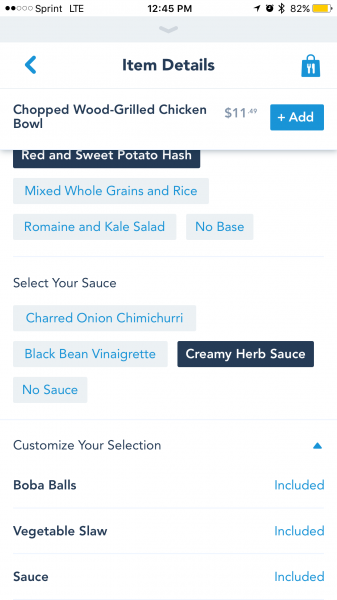Screenshot of a mobile webpage for placing a food order. The interface features black text on a white background, accented by blue highlights. At the top, the page is labeled "Item Details" beside a shopping bag icon with a fork and knife inside. The main item ordered is a "Chopped Wood Grilled Chicken Bowl" priced at $11.49. 

Customization options are displayed, starting with a choice of side dish: Red and Sweet Potato Hash, Mixed Whole Grains and Rice, Romaine and Kale Salad, or No Base. The selected option is Red and Sweet Potato Hash. Next, the sauce selection offers Charred Onion Chimichurri, Black Bean Vinaigrette, Creamy Herb Sauce, or No Sauce, with Creamy Herb Sauce chosen.

Further customization includes additions such as Boba Balls, Vegetable Slaw, and Sauce, all of which have been included in this particular order.